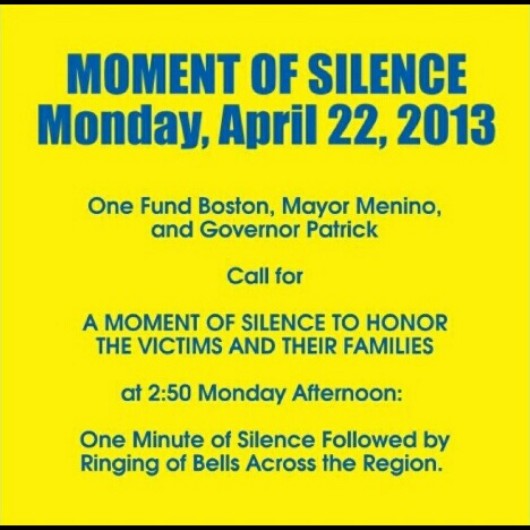The image is a vividly bright, neon yellow flyer with bold blue text. At the top, in large, bold blue letters, it reads "Moment of Silence, Monday, April 22, 2013." Below this, in smaller blue text, it states: "One Fund Boston, Mayor Menino and Governor Patrick call for a moment of silence to honor the victims and their families." Further down, it continues: "At 2:50 Monday afternoon, one minute of silence followed by ringing bells across the region." The entire design is encased within a square shape, utilizing a stark contrast between the vibrant yellow background and the striking blue font.